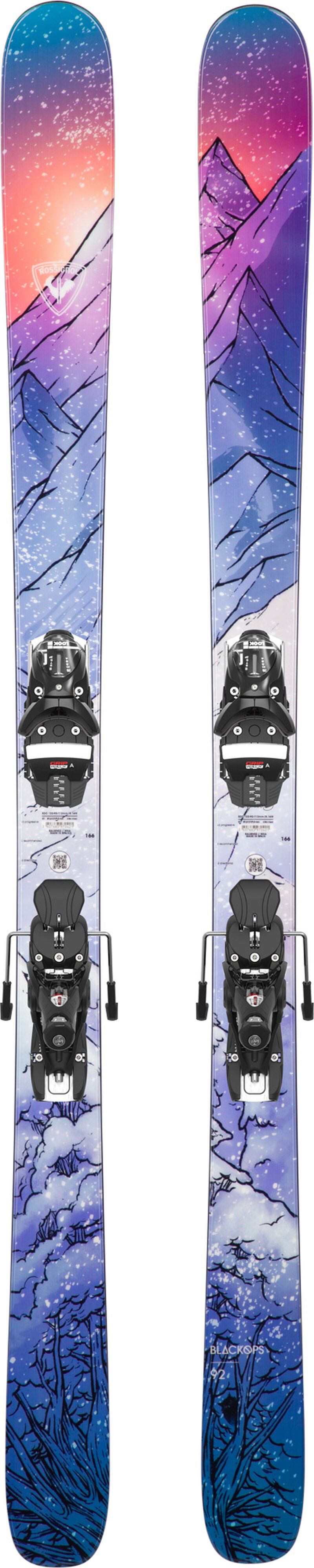The image features a detailed, cartoon-like design of a pair of custom-made skis seen from above. These skis showcase a unique mountain motif that spans across both skis, creating a symmetrical visual when placed side by side. The mountain design, hand-drawn in vibrant shades, transitions from a deep indigo blue at the bottom to a lighter blue, and then to a striking purple. The mountain peaks in purple with a gradually transitioning sky that includes hues of orangish-red and blue. 

Below the mountains, the design includes rocky elements and a few silhouette-like trees, contributing to the natural theme. The bindings, which are black with white stripes and dot patterns, are prominently placed on each ski, indicating where ski shoes would be attached. These colorful and artfully crafted skis do not bear any lettering or text, focusing solely on the exquisite and intricate artwork that makes them appear almost animated.